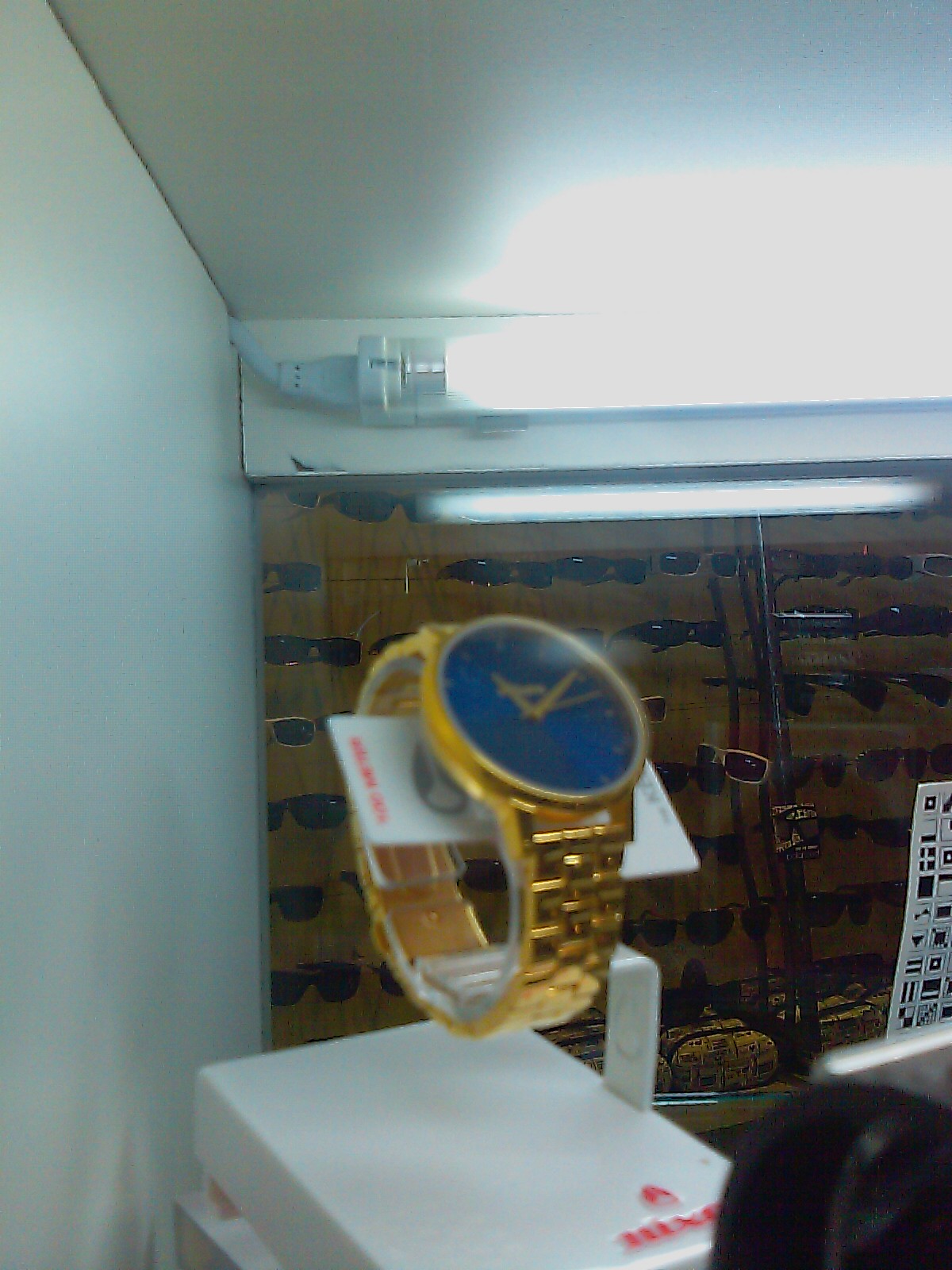In the foreground of this image, a bright gold watch is prominently displayed on a white rectangular stand, which appears to be made of plastic with additional metal components for support. The watch features a large dark blue, almost black face, highlighted by gold hour, minute, and second hands, as well as gold detailing around the edges. The face is covered by shiny glass, reflecting a bright white fluorescent light mounted toward the ceiling. This light source illuminates the watch, adding a glossy shine. The watch band is likely flexible, designed to fit securely on the wrist. Behind the watch, a white card, though out of focus, suggests branding or additional information, marked with red lettering and possibly other symbols.

In the far background, the image reveals a display of various styles of sunglasses, arranged in several rows and suspended on clear plastic hangers. The sunglasses are set against a light-colored wood surface, which appears varnished and adds a natural texture to the background. Above the sunglasses display, a power cord extends from the left wall to the ceiling, connecting to a long tube light that casts a soft illumination over the entire scene. The walls and ceiling surrounding the display and the light are white, but due to the lighting and possibly the photo quality, they exhibit different shades and tones, including hints of light blue and black. The overall focus of the image is slightly blurred, emphasizing the background over the main subject, yet the detailed elements of both the watch and the environment are discernible.